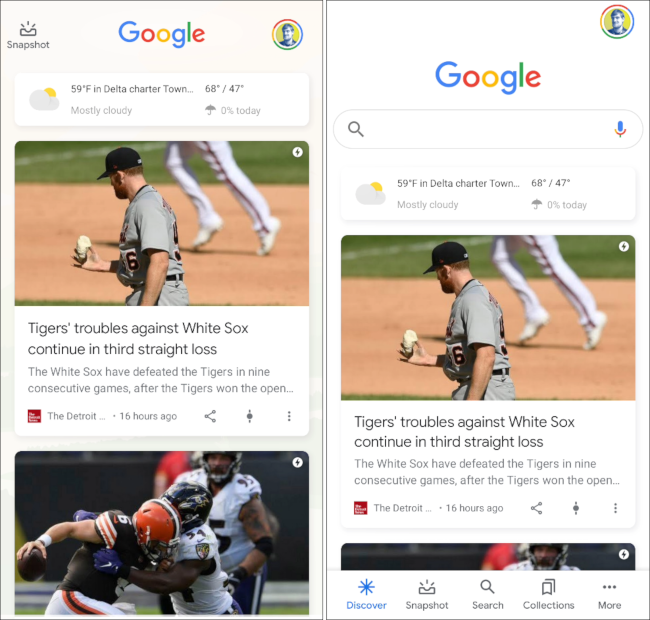A composite image composed of two screenshots captures the interface of the mobile Google search app. 

On the left screenshot:
- At the top, the recognizable Google logo, with its multi-colored letters, is displayed.
- To the right of the logo, a circular profile picture is shown, depicting a white man with brown hair wearing a black t-shirt.
- On the far left of the Google logo, a small gray phone icon is positioned with the word "snapshot" in gray text beneath it.
- Below this section, a small white rectangle presents the current weather, indicating "59°F in Delta Charter Town" alongside a cloud icon partially covered by a yellow sun. A range of "68°F / 47°F" is noted with a description "Mostly cloudy" beneath it.
- An umbrella icon follows, stating "0% today," implying no expected precipitation.
- Further below, a photograph features a white baseball player on a field, dressed in a gray uniform and a black hat. The player is holding a baseball between his thumb and forefinger.

The right screenshot is not described in this text, suggesting it might contain different or additional information that is not specified in the provided details.